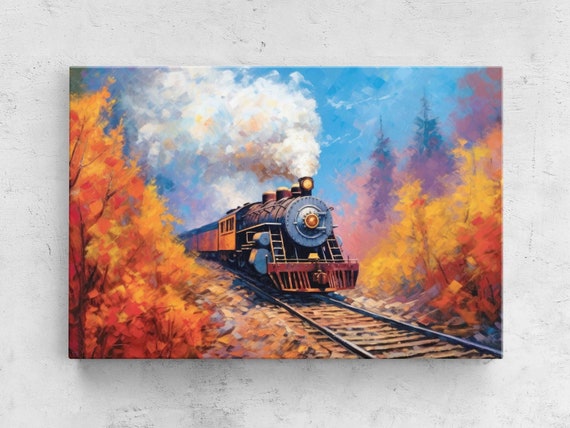Set against a white and slightly dirty wall is an illustration resembling a watercolor impressionist painting, mounted and framed. The central subject of the image is an old-fashioned train with a metallic, domed front, accurately hand-drawn to exude lifelike realism. The train is halfway through the picture, moving along tracks that angle toward the bottom right. It's emitting billowing plumes of smoke from its multiple smokestacks. Surrounding the train are vibrant autumnal trees with foliage in shades of orange and yellow, interspersed with some green trees in the background, all depicted in a softer, more impressionistic style. Above this autumn scene is a clear blue sky, contrasting with the colorful and slightly blurred leafage that flanks the train, creating a striking and dynamic composition.